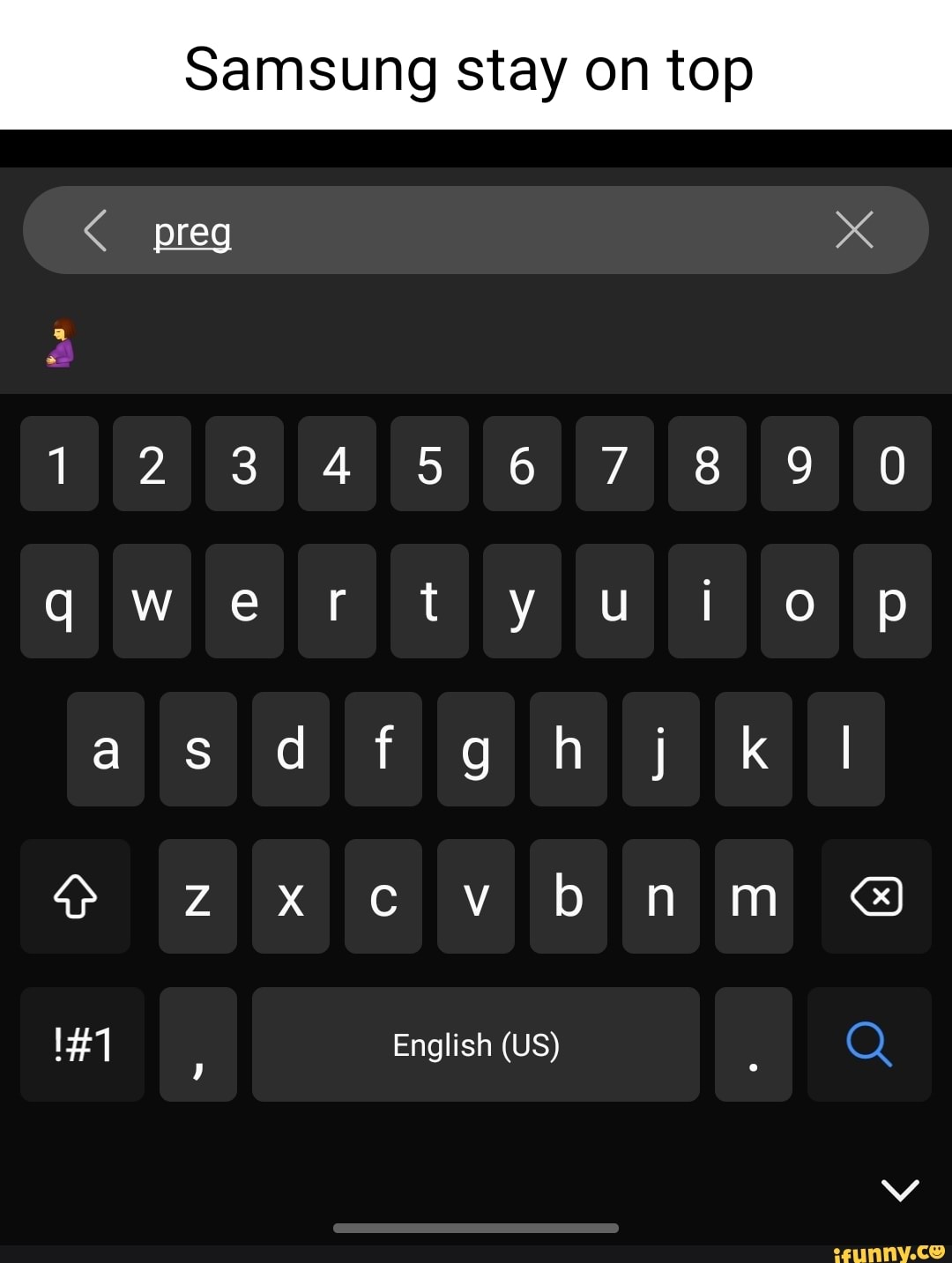The image shows a smartphone screen featuring a search bar at the top, displaying the text "preg prg," which presumably includes a typographical error. Directly below the search bar, a pregnant woman emoticon is visible. The virtual keyboard beneath it displays a standard QWERTY layout. The keys are labeled with white characters, including numbers 1 through 0 on the top row, and standard letters and symbols on subsequent rows. Special function keys such as the up arrow, backspace, exclamation point, hashtag, and comma are also visible, along with the English (US) language selector indicated by 'English (US).' Additionally, at the bottom of the screen, a down arrow and an icon for the app iFunny.co are displayed, where the 'o' in 'co' is stylized as a yellow smiley face.